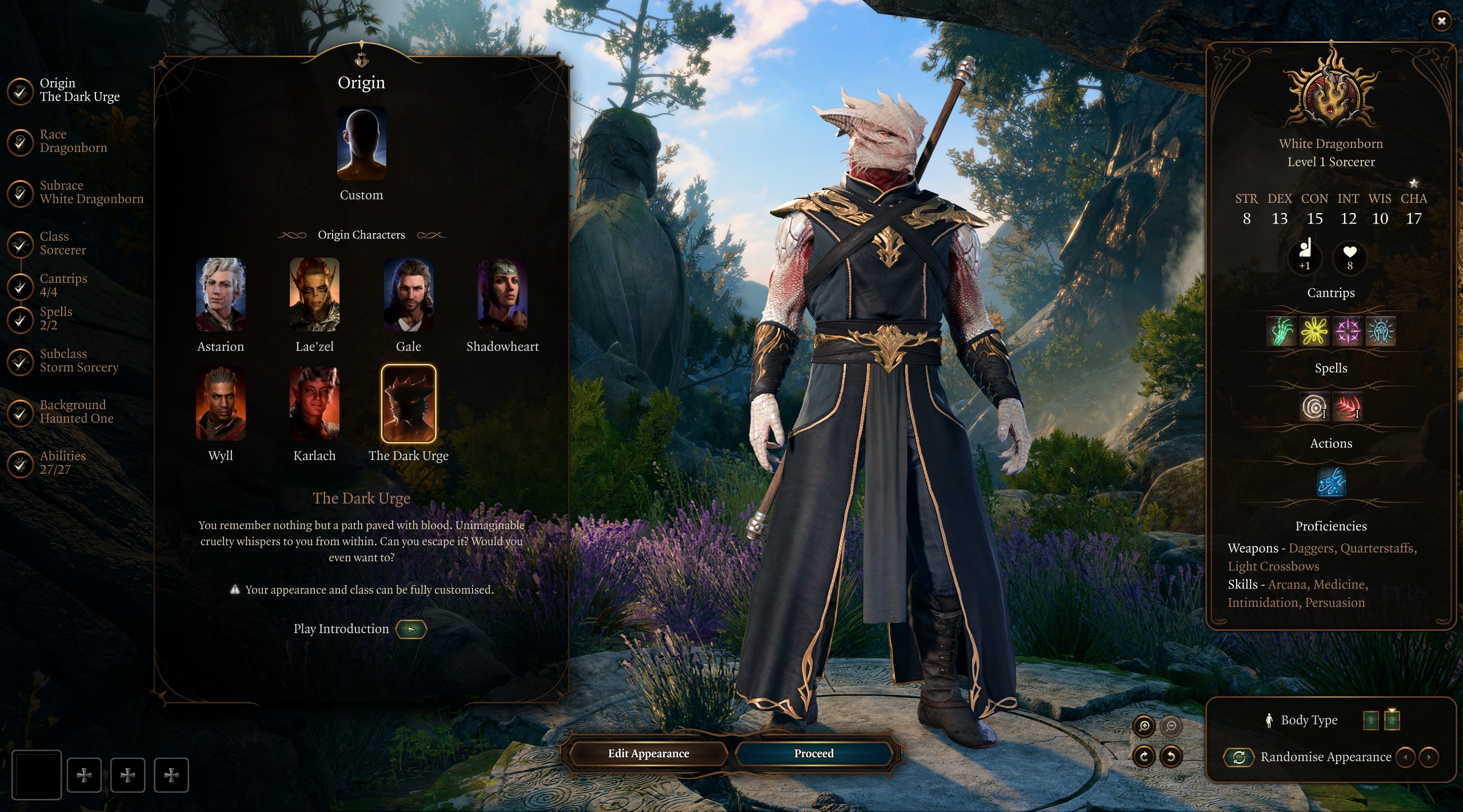The image is a still from a computer game, showcasing a character with a reptilian face, predominantly white or light gray with pinkish highlights. The character stands in the center-right of the screen, draped in a long black cloak and wearing a white headwrap. His attire features intricate gold wing-like epaulets on the shoulders, a long gray drape reaching down to the dark boots, and a black sash with golden decorations. Behind the character, the open backdrop reveals a blue sky, forest, and lavender-colored flowers, emanating an outdoor atmosphere.

Adjacent to the character, on the left side, there is a black rectangle labeled "Origin" at the top, followed by images and names of various players. Below the character, buttons reading "Edit Appearance" and "Proceed" are visible. To the right, a section consisting of numerous numbers, symbols, and words related to "Weapons" and "Skills" is displayed. The character is standing within a circular area that appears to be made of cement or granite.